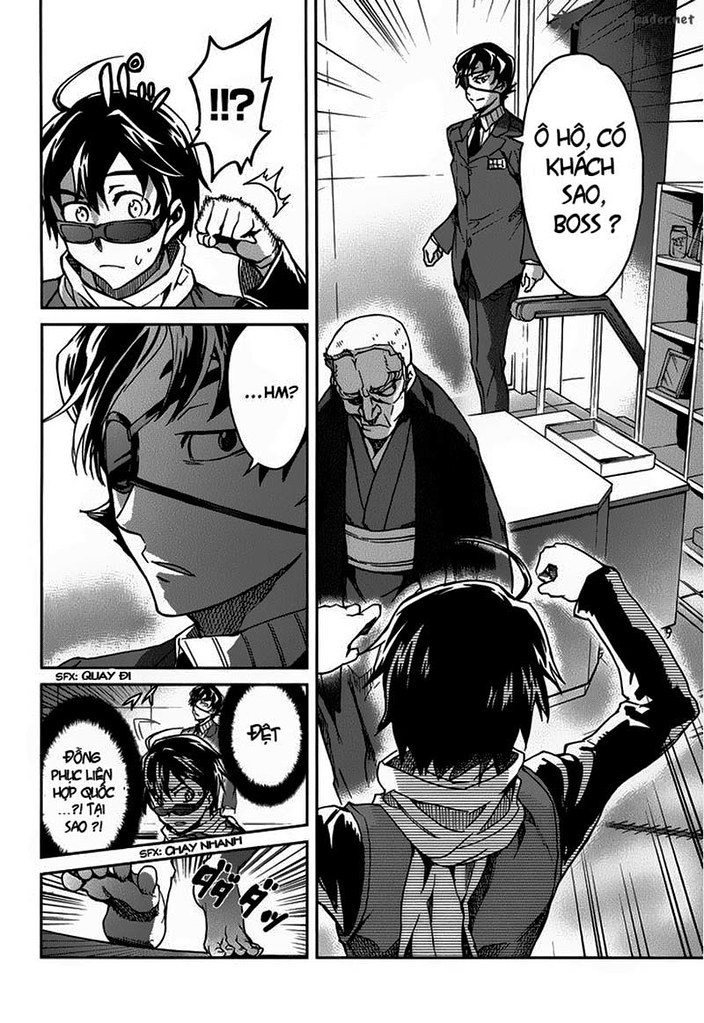The image is a detailed black-and-white anime cartoon strip consisting of five panels. The right two-thirds of the composition feature a tall rectangular panel. In this main panel, a man in a dark suit, possibly an officer, is seen ascending a staircase. He has an eyepatch and a stern demeanor, with a speech bubble next to him. Below him, another man, who appears to be elderly and dressed in a robe, stands facing the viewer. At the bottom, a man with his back to the viewer raises his right arm, showing both hands, indicating an intense moment.

On the left side, we see three stacked rectangular panels running the full height of the image. The top-left panel depicts a young man wearing sunglasses, raising his left fist, with an expression of surprise or frustration as indicated by a speech bubble with exclamation points and a question mark. The middle panel offers a close-up of the same young man, now wearing an eyepatch, with a speech bubble containing the word "hmm" to emphasize his contemplation. The bottom-left panel shows a confrontation between two men, possibly involving the same young man and another figure, with speech bubbles on both the top-left and top-right, filled with dialogue in an unspecified language. This composite illustration seems to capture a climactic moment full of tension and drama.